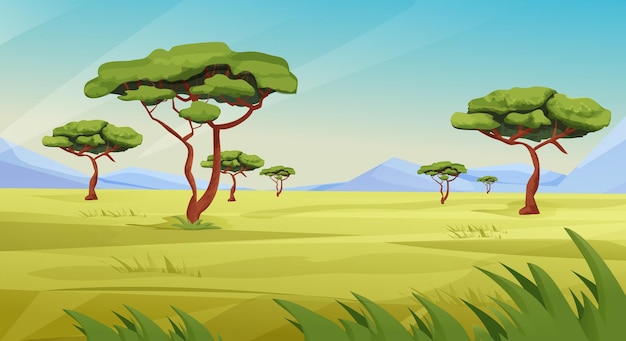This is a detailed, computer-generated cartoon image of a landscape featuring a vibrant, gradient sky transitioning from a deep blue at the top to a lighter yellowish-green near the horizon. Purple rolling hills fade into the distance, adding depth to the scene. The foreground showcases long, dark green grass, contrasting with the pale green, short grass covering the open prairie. Dotting the landscape are seven trees with gnarled, reddish-brown trunks and globes of lush green foliage atop long, sprawling branches. The trees are distributed with four on the left and three on the right, with a couple of them appearing closer to the foreground. White lines streak across the pristine blue sky, adding a whimsical touch to this serene tableau.